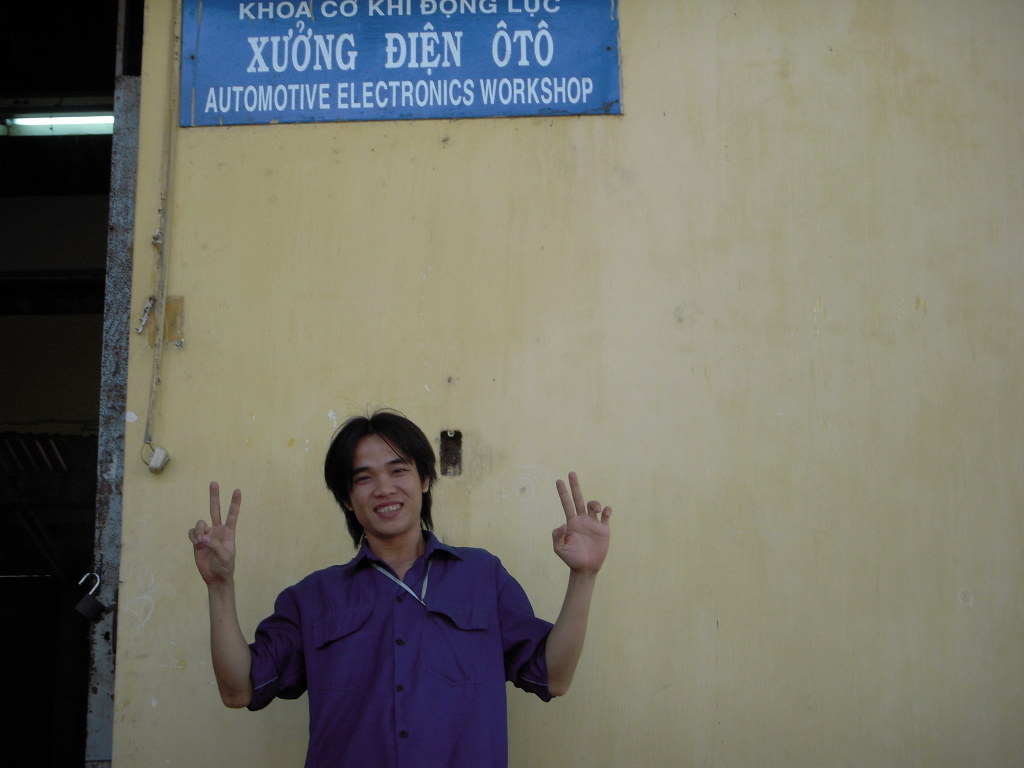The photograph appears to be taken outside of what may be a garage, indicated by the presence of a padlock on the left-hand side of the image and a silver pole above it. The backdrop consists of a wall that, though likely white originally, has become significantly dirty over time. Affixed to this wall is a blue sign with inscriptions in what seems to be either Thai or Vietnamese script. Beneath these characters, the sign reads, "Automotive Electronics Shop" in white letters. Central to the image is a young man wearing a vibrant purple shirt. He sports a short, black hairstyle and is beaming with a beautiful smile. With both hands raised, he is flashing peace signs, adding an element of joyful expression to the scene.